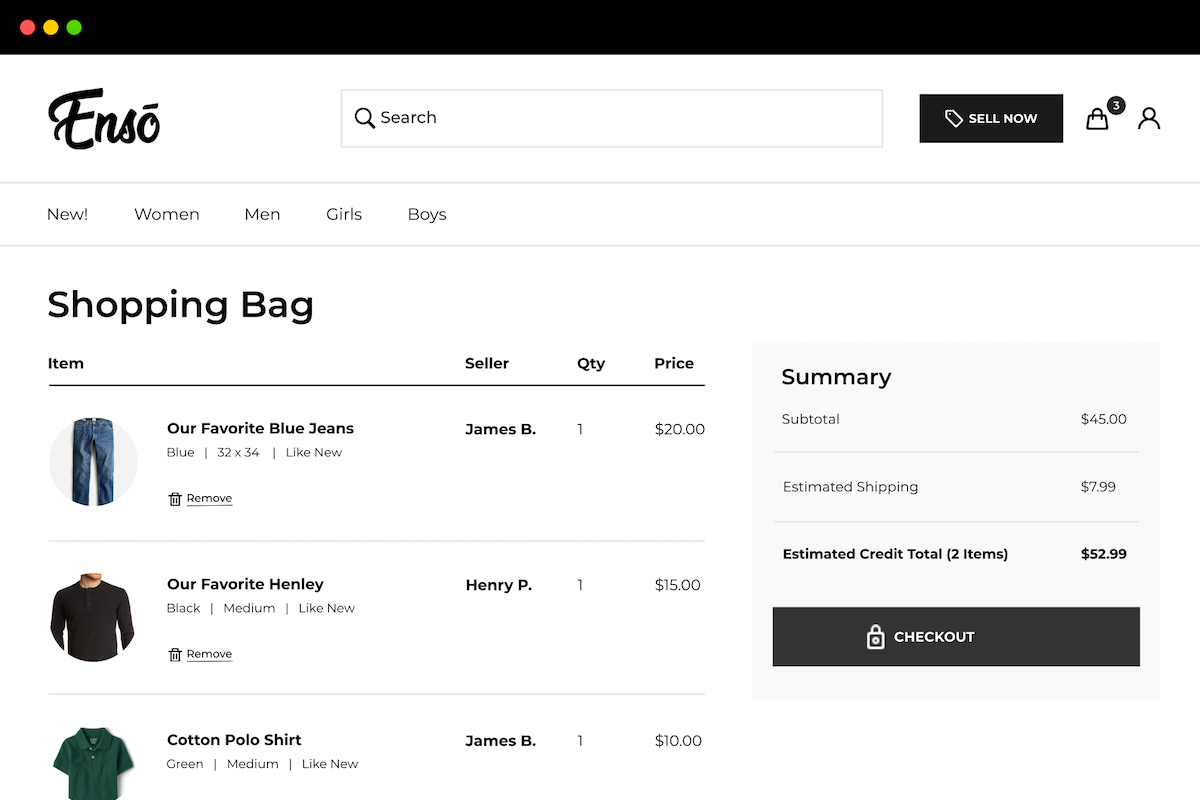The image displays a structured and detailed layout, representative of an online shopping cart or webpage. The topmost section features a black rectangle containing three small circles or dots, colored red, yellow, and green respectively. Below this, the word "ENSO" appears, with a line accentuating the 'O'.

Beneath the title, there's a gray-outlined rectangle encapsulating an icon of a magnifying glass alongside the word "search". Adjacent to this, a black rectangular tag prominently displays the text "sell now", next to an illustration resembling a purse. Additionally, a circle marked with the number "3" and a symbol indicating a person are positioned alongside.

Below these elements, a gray line precedes the words "new! women, men, girls, boys," outlined in a straightforward and categorical manner, highlighted by another subsequent gray line.

The term "shopping bag" is placed below this divider, followed by headers: "item", "seller", "QTY" (Quantity), and "price". Further details are organized in an orderly fashion: pictorial representations of various items — blue jeans, a black shirt, and a green shirt — each within circular frames. Descriptions accompany these images.

The respective sellers' names, alongside the quantities (all listed as one), and individual prices follow. A light gray rectangle beneath this area contains sections labeled "summary," "subtotal," an indistinct entry, "estimated shipping" with its corresponding price, and a financial summary of "estimated credits total" (noting two items within parentheses).

Finally, at the bottom of the layout, a prominent black rectangle featuring a lock icon is labeled "checkout," indicating the finalization point of the shopping process.